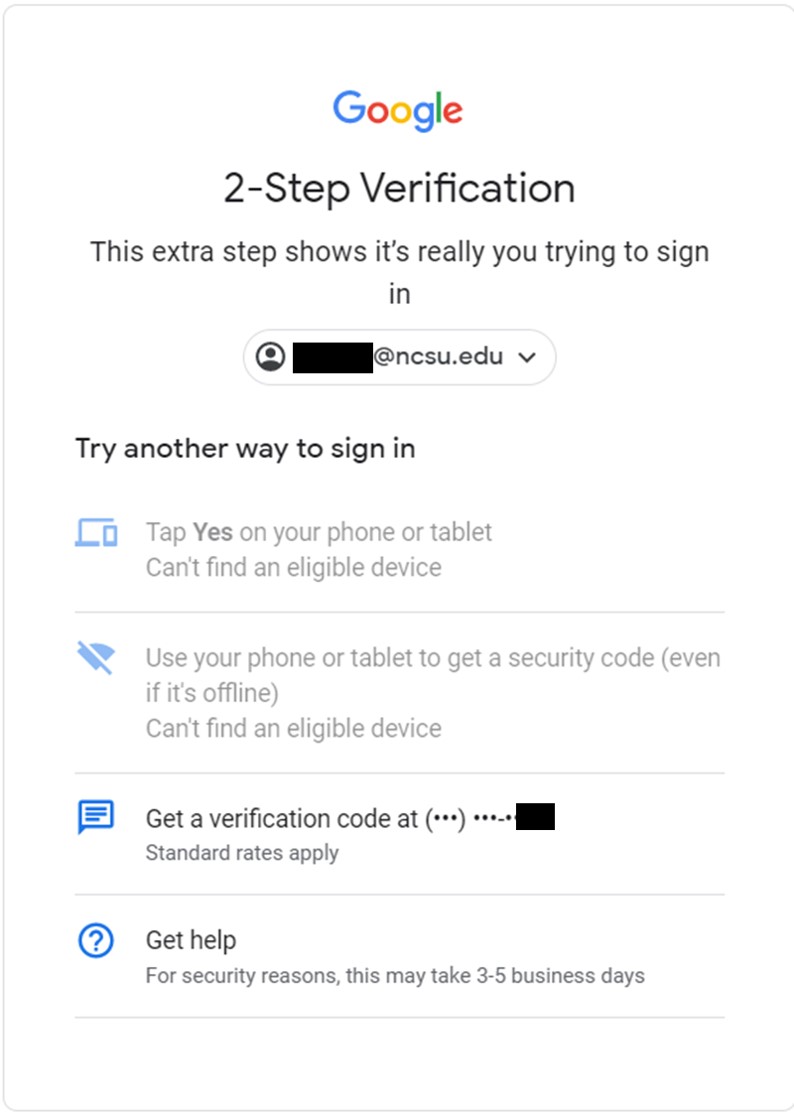The image displays Google's two-step verification process. At the top and center, the prominent and colorful Google logo is followed by the words "2-Step Verification" in black font. Beneath, a sentence reads, "This extra step shows it's really you trying to sign in." Below this sentence, an email address is partially redacted with a black rectangle to obscure some details. On the left-hand side, there are several section headings regarding alternative verification methods. The first heading, "Try another way to sign in," suggests tapping "Yes" on a phone or tablet. The next heading, "Use your phone or tablet to get a security code, even if it's offline," follows with an option to "Get a verification code at [redacted]." The final heading, "Get Help," notes that for security reasons, assistance might take three to five business days. These instructions detail various methods for completing the verification process, emphasizing that tapping "Yes" on a phone is the quickest method.